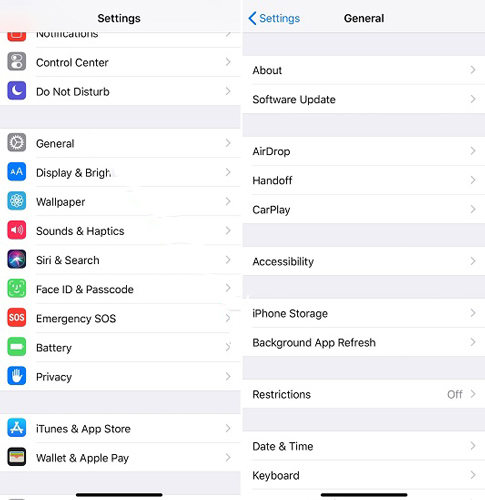The image features two side-by-side screenshots of an iPhone's Settings app displayed in Light Mode, characterized by a white background. The left screenshot shows the top-level settings menu, including options such as Control Center, Do Not Disturb, General, Display & Brightness, Wallpaper, Battery, and Privacy. The right screenshot reveals the General settings subcategories, which are accessed by tapping 'General' from the top-level menu. This screen includes options like About, Software Update, AirDrop, Handoff, CarPlay, Accessibility, iPhone Storage, and Background App Refresh, among others. The Restrictions section within General settings displays 'Off,' hinting at possible parental control features that are currently disabled. A ‘Back’ button is present, allowing users to return to the higher-level settings menu.